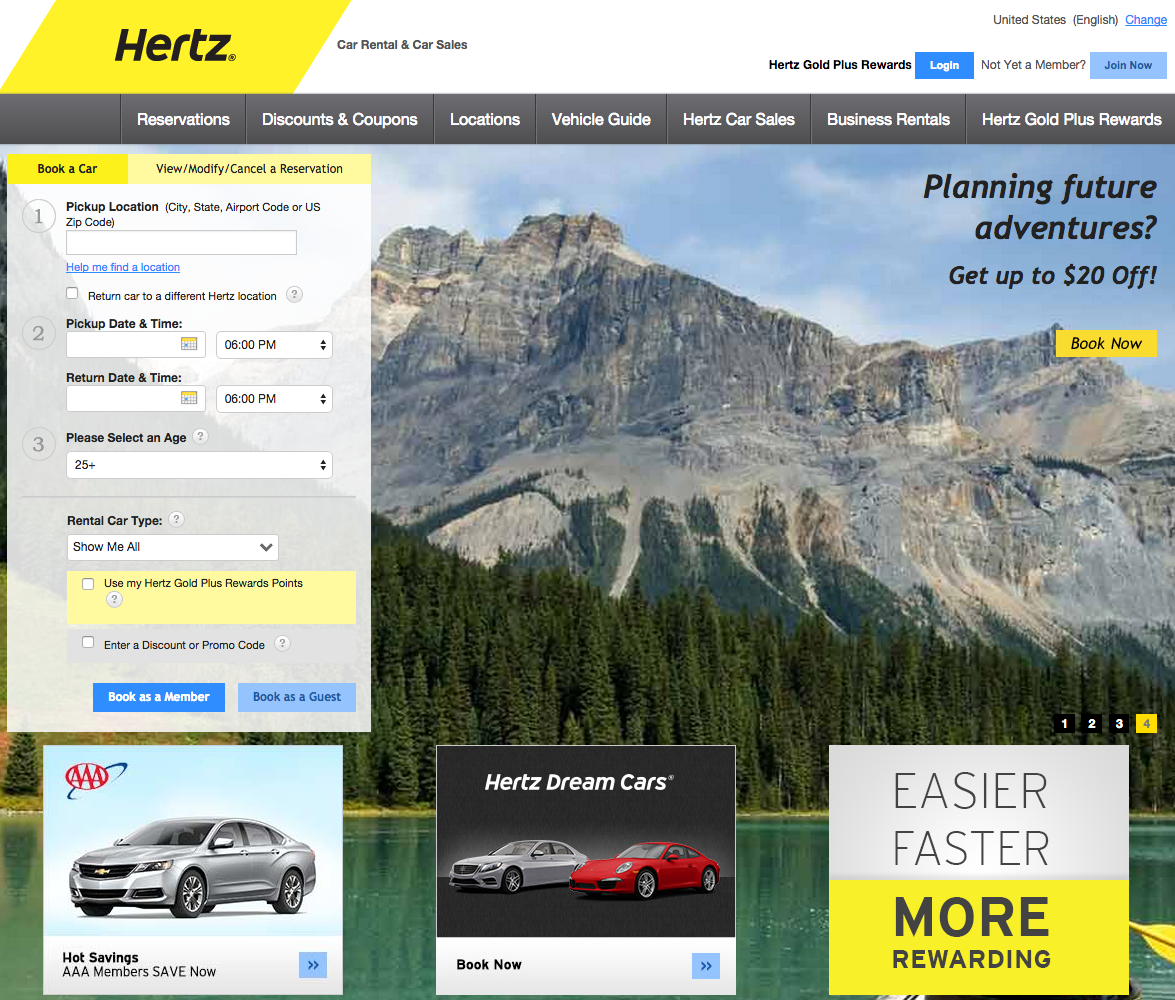The screenshot showcases the Hertz rental car homepage, brimming with detailed elements. At the top left corner, a yellow parallelogram hosts the prominent, bold black font text "Hertz." Adjacent to it, in smaller black font, the phrases "car rental" and "car sales" appear.

On the upper-right section of the header, the region and language "United States (English)" are listed, followed by an underlined "change" in blue font. Directly beneath this, the bold black text "Hertz Gold Plus Rewards" is featured in a diminutive size. Next to it, a blue box with white print reads "login." Further to the right, the small black text "not yet a member?" is adjacent to a light blue box with dark blue text that says "join now."

Below this header lies a horizontal, light gray menu bar with white font menu items, including: "Reservations," "Discounts and Coupons," "Locations," "Vehicle Guide," "Hertz Car Sales," "Business Rentals," and "Hertz Gold Plus Rewards."

Dominating the central background, an image of a serene mountain reflected in a lake sets a picturesque scene. In the top right corner of this image, black text reads "Planning future adventures? Get up to $20 off." Below this offer, a yellow rectangular button with black font prompts users to "book now." On the left side of the page, a form is available for visitors to fill out to rent a car.